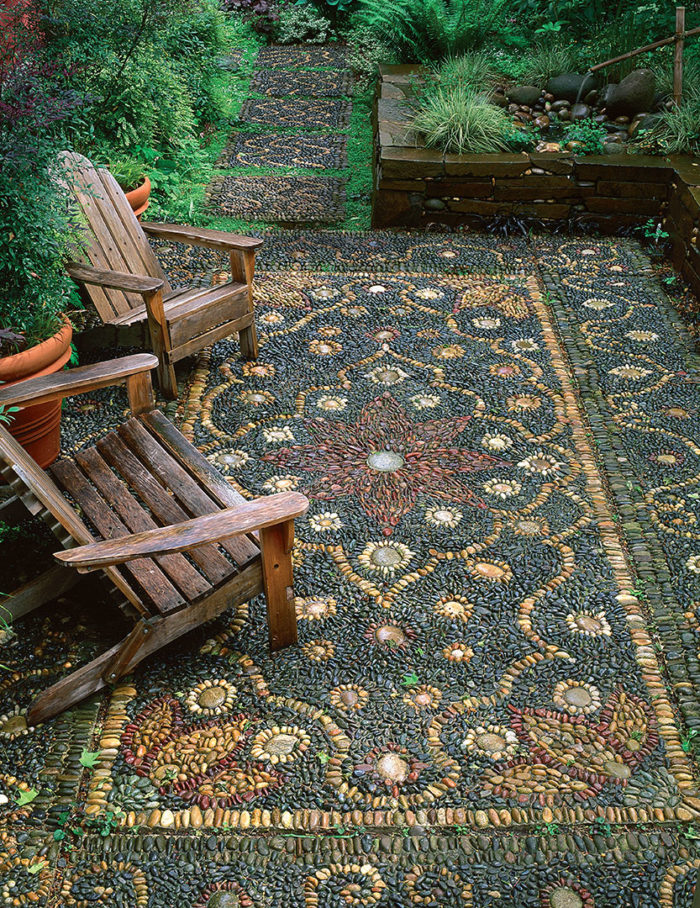The photo captures an intricately designed outdoor patio resembling a serene botanical garden setting. At the center of attention is a stunning rock sculpture that mimics the appearance of an ornate oriental rug, meticulously crafted from countless small stones. The "rug" showcases an elaborate medallion pattern, with vibrant shades of red, blue, yellow, and green stones forming a central red flower. This artistic arrangement is complemented by raised brick planters filled with lush greenery and various plants, contributing to the garden ambiance.

Flanking the stone artwork are two laid-back wooden Adirondack-style chairs with high backs, offering a perfect spot to enjoy the outdoor haven. Between the chairs sits a large, decorative clay planter, adding to the patio's charm. A pathway meanders through the backyard, bordered by additional planters and rich plant life, enhancing the tranquility and inviting atmosphere of this meticulously crafted outdoor space.